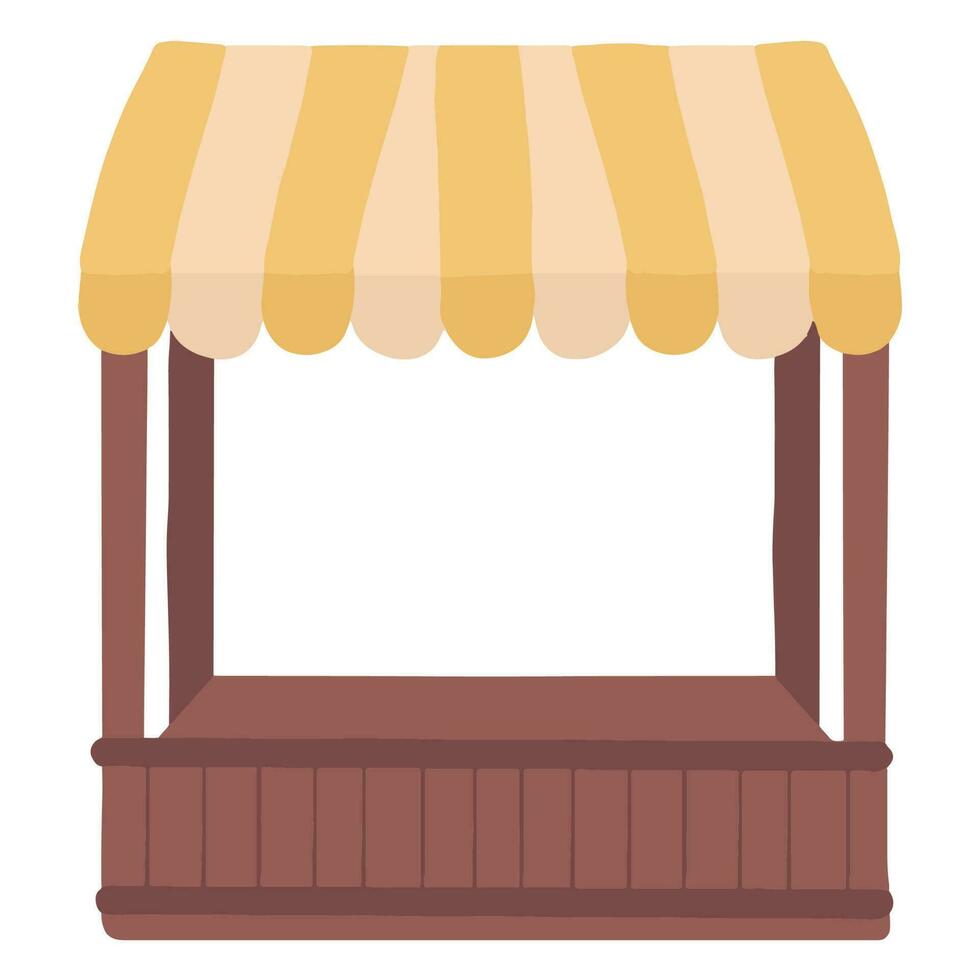The image is a computer-generated drawing of a simple brown platform with slatted boards forming its base. The platform features a raised wooden barrier around its edge and is covered by a tent-like canopy with legs on each side. The canopy's sunshade is striped with alternating colors, predominantly dark yellow, light yellow, green, and possibly a mix of orange and peach hues. The background of the image is white. The booth, devoid of any personnel, appears to be designed for display purposes, with no visible stairs for access, hinting they might be located at the back, out of sight.